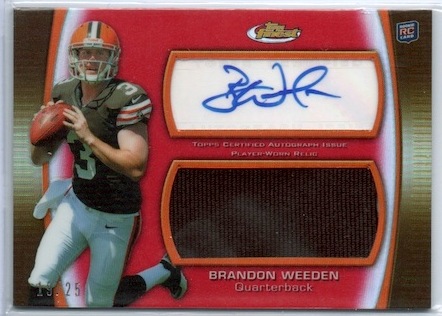This color photograph in landscape orientation showcases a commemorative football card encased in a protective plastic sleeve. The card features a dynamic image of Brandon Whedon, a white man, captured in a running position wearing a Cleveland Browns uniform. He dons a brown jersey with white and red stripes on the sleeves, the number three prominently displayed, white Nike pants, and an orange helmet with brown and white stripes. Whedon holds a football tightly against his chest. The background of the card is visually striking, featuring a gold backdrop with a red semi-circle and what appears to be Venetian blinds behind him.

Above Whedon, in a white rectangular panel, is his autograph in blue ink, marked by text reading "Topps Certified Autograph Issue Player Worn." Below this, a black panel displays the player's name and position: "Brandon Whedon, Quarterback." At the very top, another white panel likely indicates the brand, inscribed with "Topps Finest" or "Topps Football." Additionally, the card bears the "RC" logo on the bottom right, signifying a rookie card, and has a watermark reading "19.25" in the bottom left corner. This detailed card blends photographic representationalism and product photography, visually encapsulating the essence of Whedon's professional image.